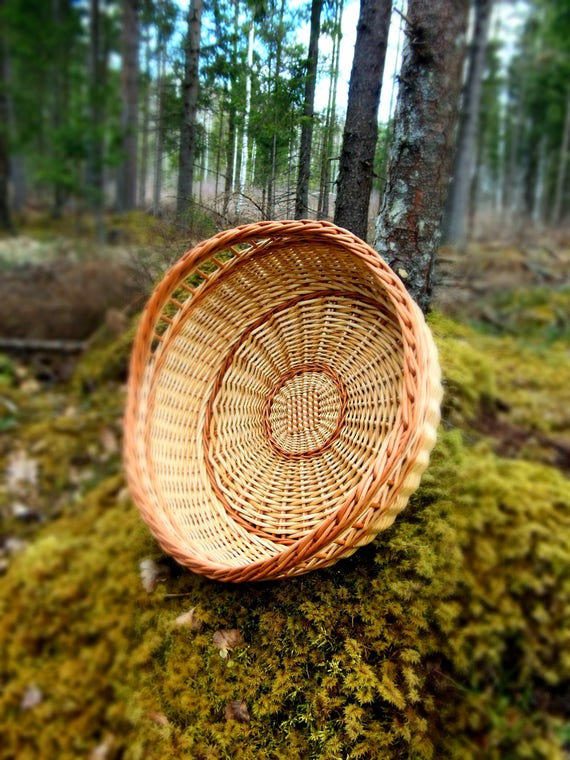This is a close-up shot of a large, light-tan woven basket intricately braided along the rim, sitting on its side on a vibrant, green moss-covered forest floor. The basket, which is empty, is positioned slightly left-of-center in the photograph and faces the forefront. The forest bed is entirely carpeted in moss, creating a serene green blanket under the basket. In the background, there's a blur of tall, slender trees and a hint of blue sky peeking through the foliage, conveying a sense of depth and seclusion. To the left, a fallen log lies slightly out of focus, adding to the natural setting. One tree in the foreground stands out with distinct bark, juxtaposed against the otherwise blurred backdrop of dense forestry, emphasizing the basket's placement in the tranquil forest scene.